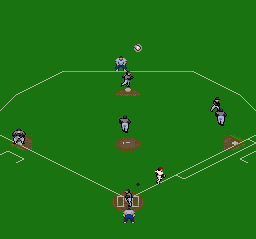This square image showcases a scene from a minimalist video game, set against a solid green screen that depicts a baseball diamond. The bases and the pitcher's mound are marked in brown, adding a touch of contrast to the scene. The simplicity of the design is evident in the characters, which are outlined in black and lack intricate details. The baseball diamond is represented by a series of yellow dotted lines. In the scene, one player is seen running from the batter's area towards the first base. On the right side, additional players and the pitcher are visible, with their backs to the viewer, enhancing the game's straightforward aesthetic.